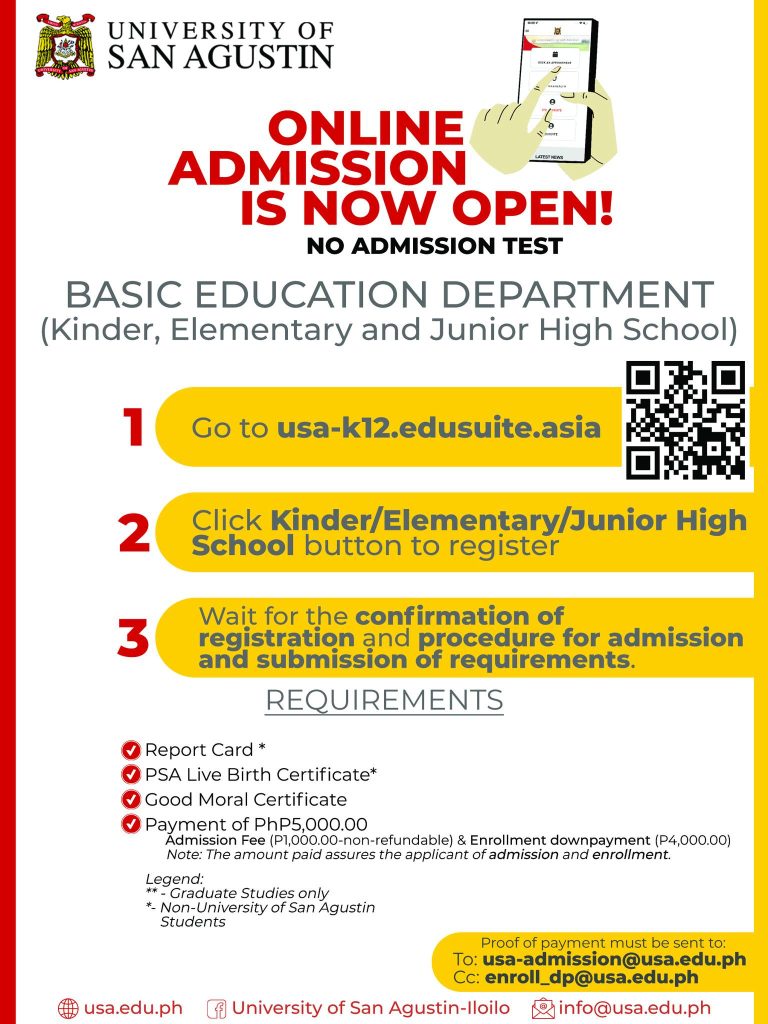This image appears to be an advertisement from the University of San Augustine. The design is split by a thin vertical bar: a red bar on the left side and a yellow bar on the right.

In the upper left corner, there is a crest or logo of the university. To the right of the logo, the text reads, "University of San Augustine." Beneath this, the word "Online" is prominently displayed. Below the text, an image shows hands holding a phone, likely indicating online activity.

The central message of the advertisement is: "Online admission is now open. No admission test required for the Basic Education Department." This department covers Kinder, Elementary, and Junior High School levels.

Towards the center-right of the advertisement, there is a QR code available for further action. Below this, three steps are listed for the admission process:
1. Go to the website.
2. Click on a specific section.
3. Wait for confirmation of registration and proceed with submission of requirements.

At the bottom of the image, there is a list of the necessary admission requirements followed by contact information for further assistance.